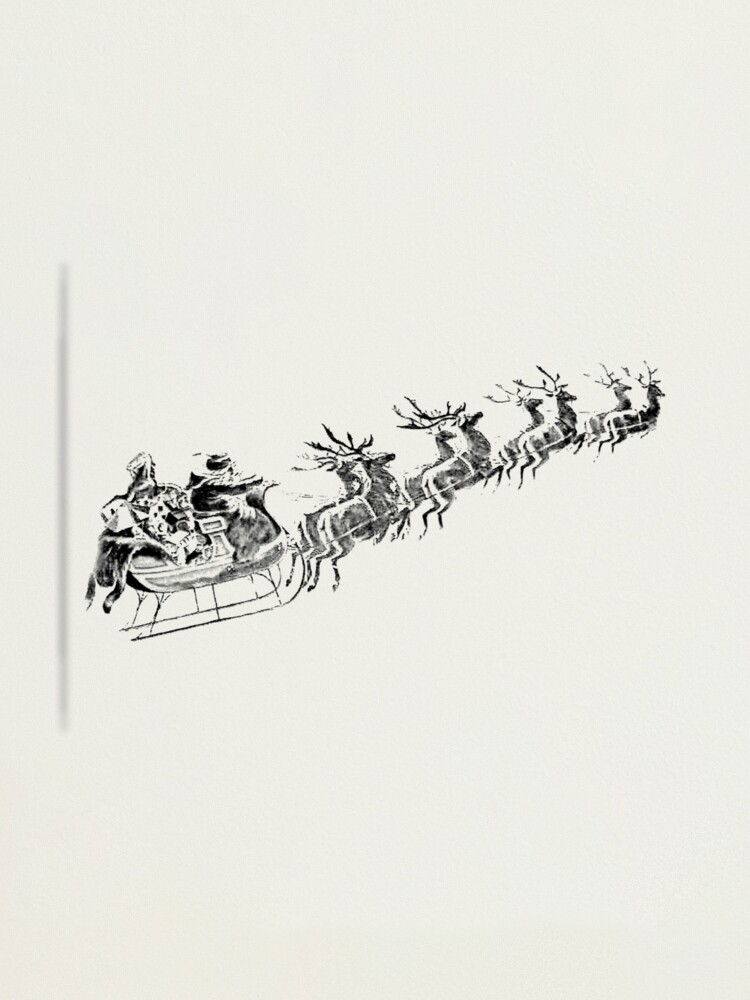This black and white illustration, resembling a 1950s children's book style, features Santa Claus in his sleigh loaded with toys, being drawn by eight reindeer arranged in four pairs. The sleigh is depicted flying off towards the right corner of the image, with the reindeers complete with antlers. Santa is seated at the front of the sleigh, though his facial features are not visible, only the outline of his clothing. The sleigh's runners curve upwards at the front. The backdrop is a plain, off-white or cream-colored piece of paper, with a faint gray vertical line approximately seven to eight inches long on the left-hand side of the image. This detailed illustration is centrally placed on the paper, making it the focal point and possibly suggesting it could be a stamp.